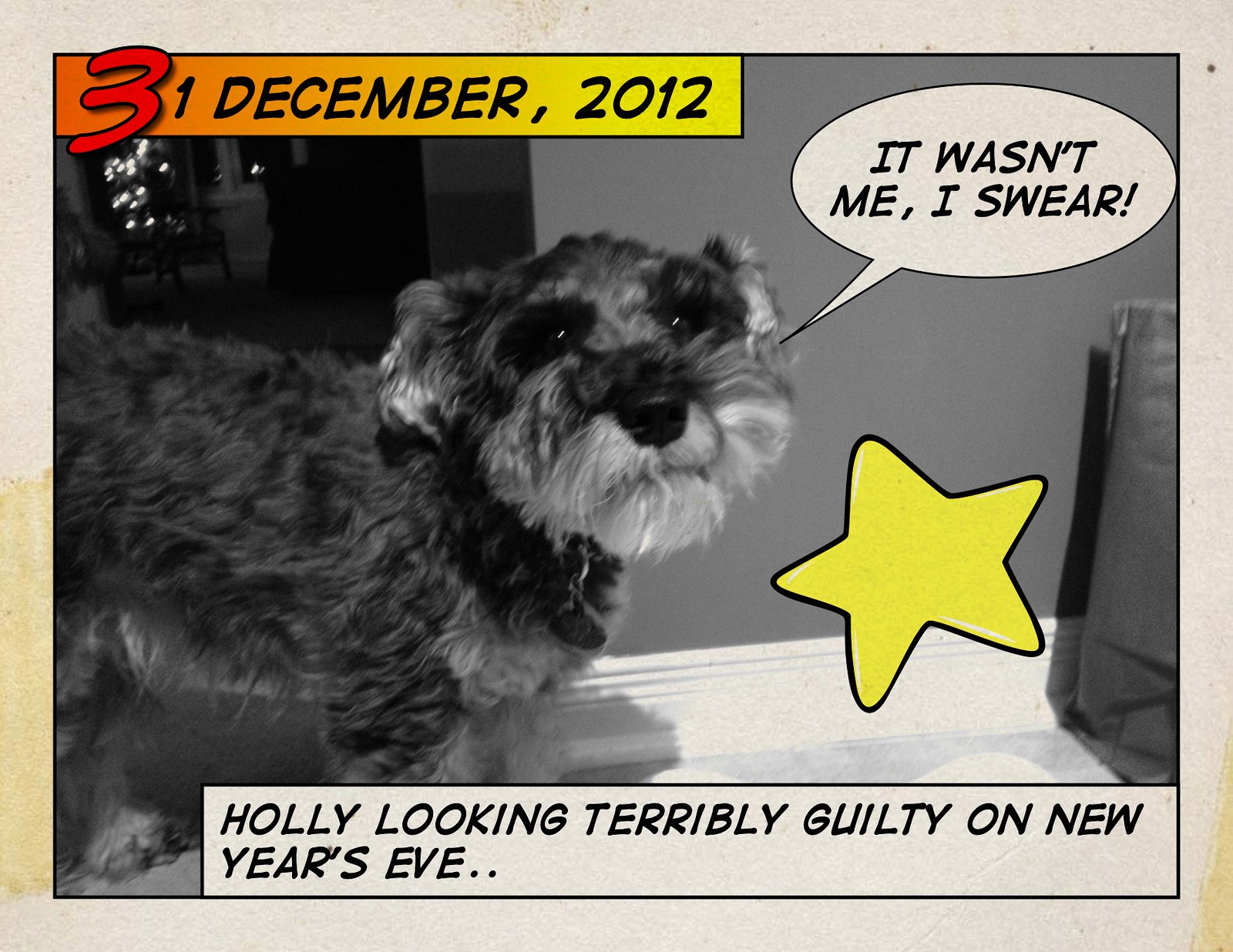The image portrays a postcard featuring a black-and-white photograph of a Mini Schnauzer dog with a puzzled expression, looking directly at the viewer. A comic-style filter enhances the playful appearance of the image. The background is a gradient of gray to black, with an out-of-focus Christmas tree visible in the far left corner. The card is approximately five inches tall and six inches wide, with an off-white border marred by yellow stains on the left-hand side and lower right corner. The photo itself is framed by a thin black pinstripe. 

In the upper-left corner, there's a rectangular banner that transitions from orange to yellow, bearing the date "31 December, 2012" in large orange and black numbers. A white thought bubble with black text emerges from the dog's mouth, declaring, "It wasn't me, I swear." Just beneath the text bubble, a yellow star with a black outline accentuates the playful theme. At the bottom of the card, a white rectangle with black text reads, "Holly looking terribly guilty on New Year's Eve," adding a caption to the dog's innocent yet guilty expression. Overall, the postcard charmingly encapsulates a whimsical and humorous moment on the eve of the New Year.